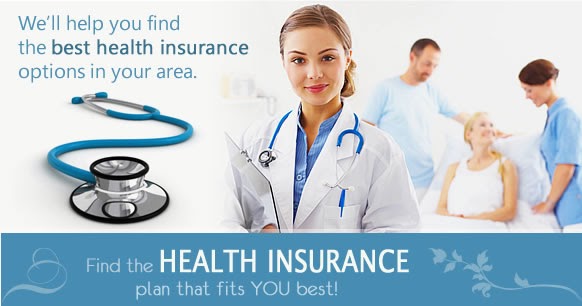A promotional image showcases a young woman with light brown hair and pink lipstick, wearing a white lab coat over a blue button-up shirt, with a blue stethoscope draped around her neck. She holds a clipboard and has a slight smile on her face. In the background to the right, another young woman with blonde hair is seen lying in a hospital bed, smiling brightly at two people dressed in blue shirts beside her. One is a young woman with brown hair, and the other is a man, likely in his 30s or 40s, with brown hair. The upper left corner of the image features text stating, "We'll help you find the best health insurance options in your area," accompanied by a blue stethoscope icon. A blue banner adorned with subtle floral designs runs across the image, bearing the message, "Find the health insurance plan that fits you best." The words "health insurance" are prominently displayed in a large, bold white font, as is the phrase "best health insurance" in the upper portion.